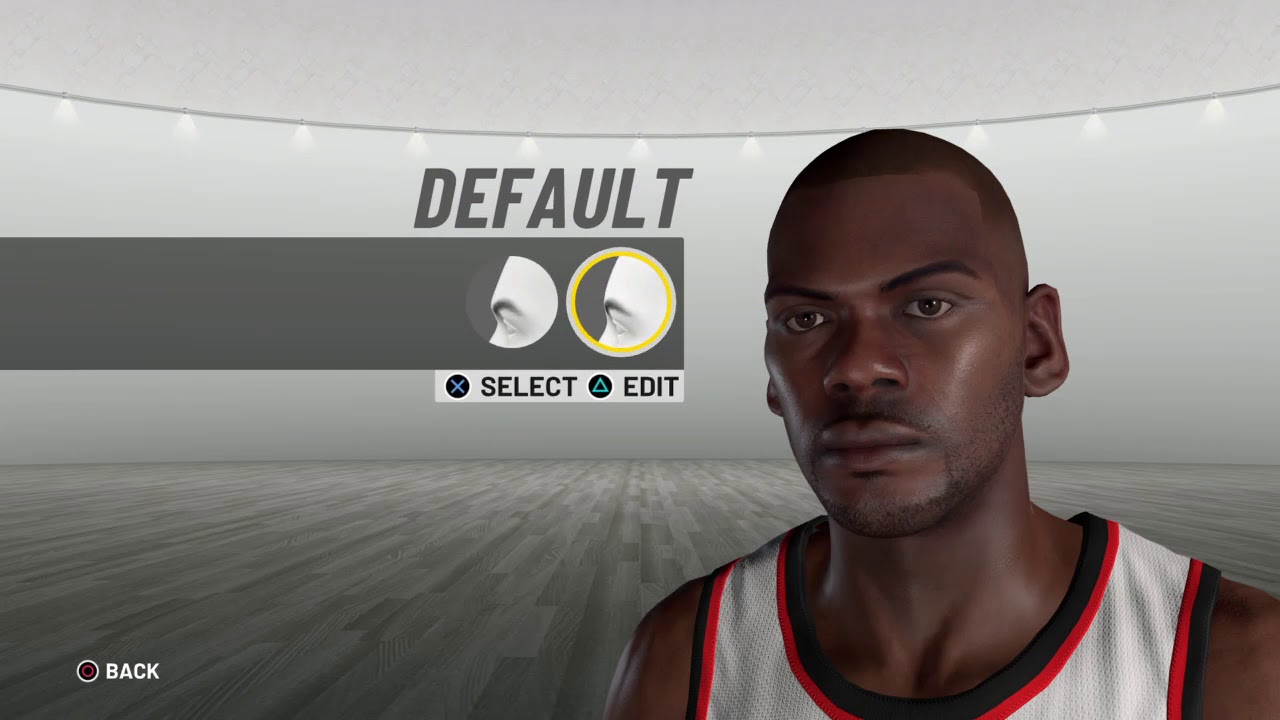The image is predominantly gray and rectangular in shape, featuring a young man with closely shaved hair, a mustache, and a light short beard positioned on the right-hand side. He is wearing a white basketball jersey adorned with an orange line around the shoulders, armpit area, and collar. Above his head, a string of white light bulbs is draped in a slightly sagging manner. These elements appear to be from a video game's character optimization window, indicating that the figure is a virtual avatar, not a real person.

The center of the image displays the word "DEFAULT" in dark gray letters beneath the string of lights. Entering from the left side of the image and extending halfway to the center is a large gray banner. This banner features a side profile view of eyebrows on the left side of a white dummy face within a circle. The circle on the right of this banner is circled in yellow, indicating it has been highlighted.

Below the highlighted circle is a gray bar with a gray circle on the left that contains a blue "X." To the right of this circle, in black text, the word "SELECT" is written. Adjacent to this, on the right-hand side against the gray background, is a blue triangle inside a gray square with the word "EDIT" written beside it.

In the bottom left corner of the image, a button outlined in white and red reads "BACK" in bold white letters.